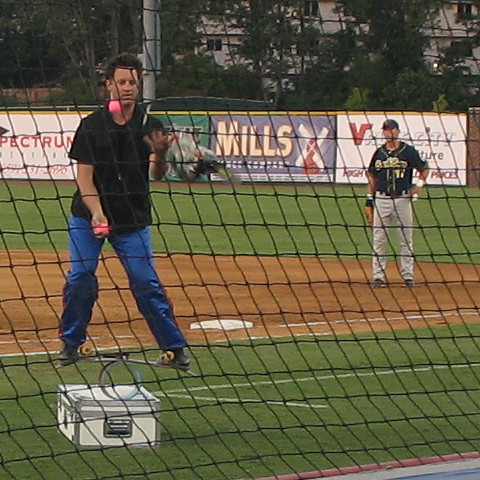This digital photograph, taken outdoors, captures a lively scene on a baseball field with a green outfield and a dirt ground in the foreground. Dominating the background is a white, at least two-story building partially obscured by very dark trees. Along a wall with advertisements, one banner reads "Spectrum" in gray font, another says "Mills" in yellow font alongside a red windmill with white blades, and a third displays "Value City Furniture," with a red "V" and the rest of the text outlined in black on a white background. 

In the foreground, close to the camera, the neatly cut grass frames two distinct individuals. On the right stands a baseball player dressed in a black shirt, gray pants, and a baseball cap, looking directly at the camera. Slightly closer, a man seems to juggle two pink balls mid-air while wearing a black short-sleeved dress shirt and blue jeans. A white box with silver edges rests on the ground in front of him. A black net extends across the lower part of the image, completing this vivid portrayal of a moment captured on the baseball field.